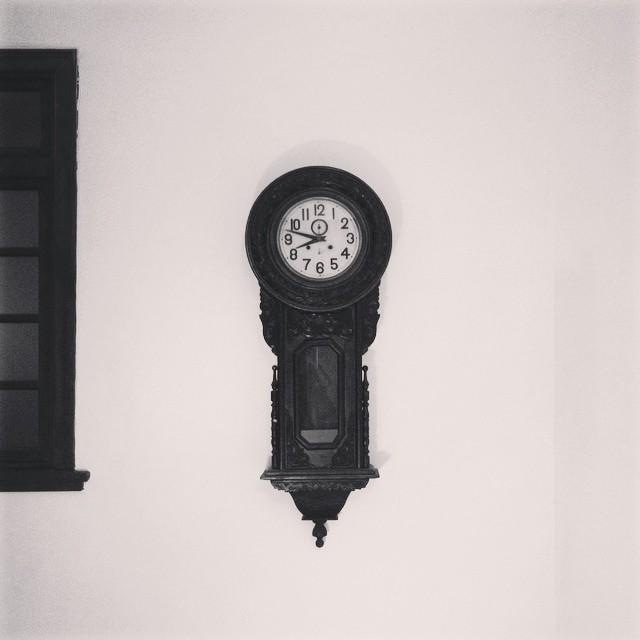This detailed photograph depicts an ornate black grandfather clock mounted on a stark white wall. The top portion of the clock features a round, white clock face with large, bold black numbers ranging from 1 to 12, clearly visible in an easy-to-read font. The clock shows a time of approximately 8:47. Both the minute and hour hands are black, adding to the clarity against the white background. Below the 12, there is a smaller, circular inner clock, though its specifics are indistinguishable. The clock's face is encased within a black circular frame, extending down into a taller, rectangular section with a glass window, presumably displaying the pendulum. There are two black circular elements located above the 4 and 8, contributing to the ornate detailing.

The clock body, made of dark wood, has a rich texture and is adorned with curvaceous dowels on the sides, narrowing to a decorative point at the bottom which resembles the posts of a bed frame. The clock casts a dark shadow on the white wall, giving depth to the image. On the left edge of the photograph, part of a black bordered window with horizontal dividers is visible. The window is dark-tinted, and nothing outside can be seen through it. A hint of dark gray or black cabinetry is also visible to the left, adding further context to the setting. The overall photograph has a monochromatic aesthetic, enhancing the intricate details of the grandfather clock against the plain background.